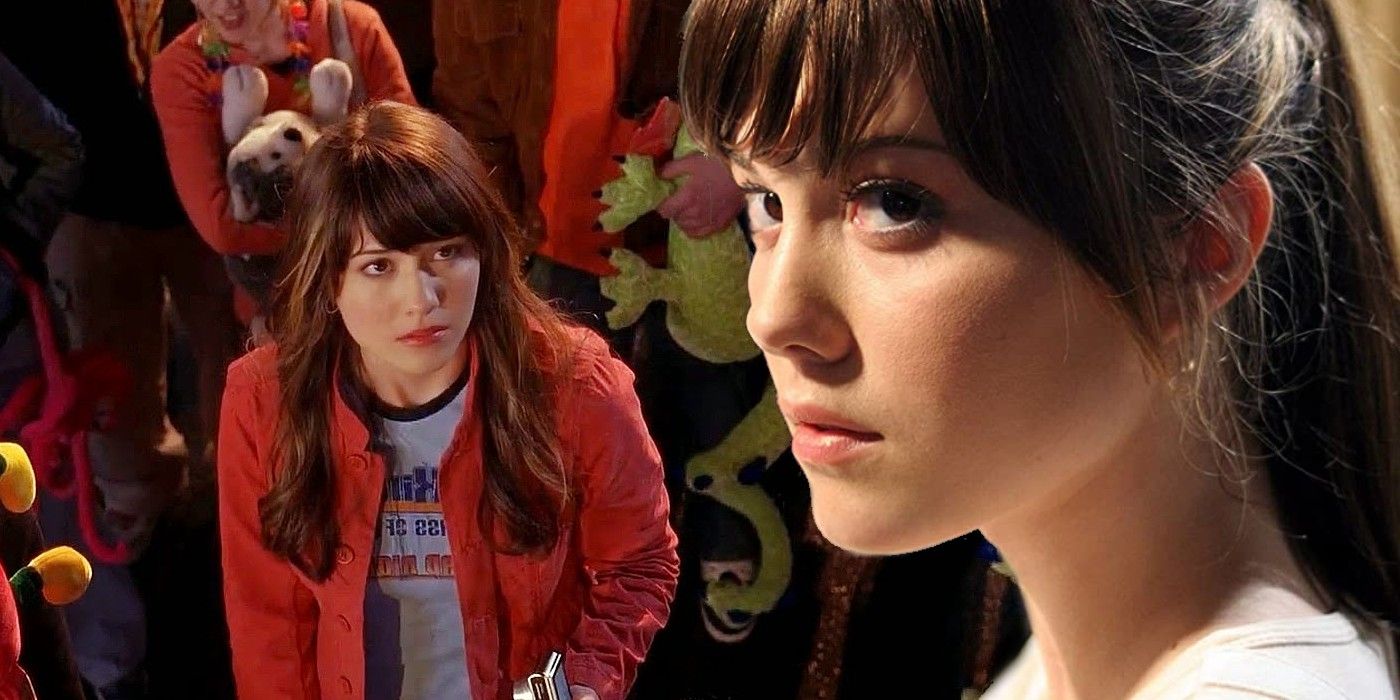The image appears to be a detailed still from a movie or television show, possibly from the 80s. In the foreground, on the right side, a young woman with fair skin and dark brown hair styled in bangs and a ponytail is captured in a close-up, looking slightly to the side. She wears minimal makeup and a white shirt. On the left side, another young woman, potentially the same person, has long, wavy, reddish-brown hair with bangs. She is dressed in a red jacket over a gray t-shirt with indiscernible writing, and she appears to be looking at the first woman while holding a camera.

In the background, there are indistinct figures contributing to the scene's depth. One individual is partially visible, holding a stuffed husky toy. Another person behind the young woman with the ponytail is holding a stuffed dragon or lizard. The overall atmosphere and styling suggest an 80s aesthetic, adding a nostalgic feel to the image.